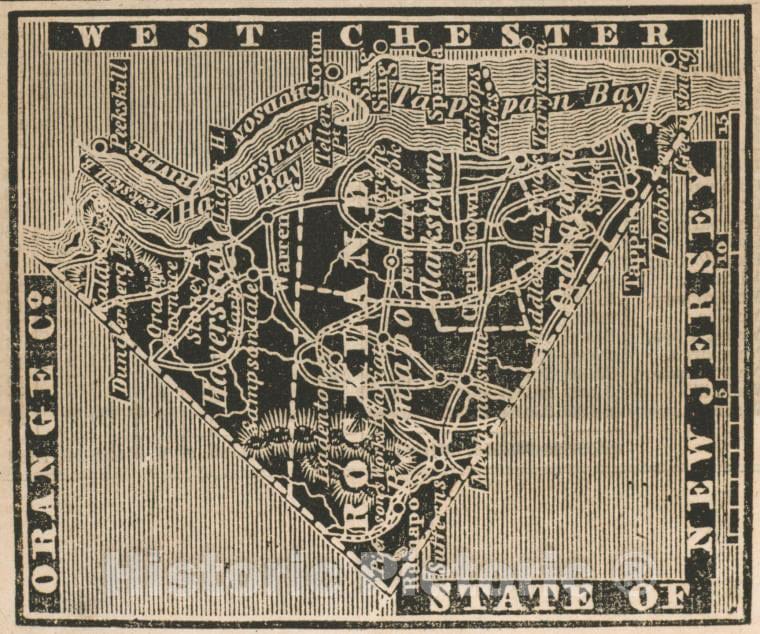This is an image of a historical map, likely an old ink block print, characterized by its black-and-yellow color scheme due to the paper's yellowing with age. The map is contained within a V-shaped or upside-down triangular boundary and features a mix of legible and intersecting, hard-to-read text. The top of the map reads "Westchester," while the bottom right extending upwards says "State of New Jersey," then "Orange Co." on the left upward side. Prominent map features include Haverstraw Bay, Tappan Bay, Peekskill, and the city of Rockland, with waterways and homes labeled throughout. The text "Rockland" is visible running sideways in the center of the triangle. Additionally, there is a faint historic watermark, potentially reading "historic pictory," adding to the map’s antiquity and character.